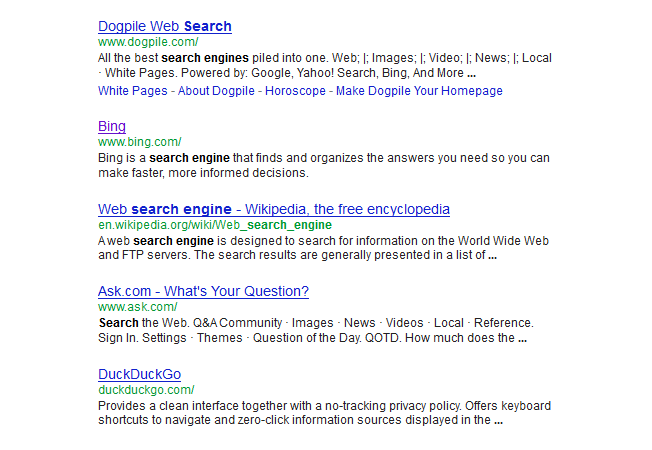The image depicts a webpage from Dogpile Web Search, accessible at www.dogpile.com. At the top, the website showcases its tagline, "All the best search engines piled into one," and provides navigation options labeled as Web, Images, Videos, News, Local, and White Pages. The search functionality is powered by major search engines including Google, Yahoo, and Bing. Below this header, the first search result listed is for Bing, highlighted in purple, indicating it has been visited. The URL www.bing.com is displayed in green, alongside a description stating, "Bing is a search engine that finds and organizes the answers you need so you can make faster, more informed decisions."

Further down, another search result is presented in blue for Wikipedia, under the title "Web search engine - Wikipedia, the free encyclopedia." The green URL leads to the detailed entry on Wikipedia, explaining that "a web search engine is designed to search for information on the World Wide Web and FTP servers. The search results are generally presented in a list..."

Following the Wikipedia entry, there is a result for Ask.com, highlighted by the phrase "What's your question?"

At the bottom of the search results, DuckDuckGo is listed with its URL, duckduckgo.com, and accompanying information about the search engine. The clean layout and organization demonstrate Dogpile's aggregation of various search engine results into one convenient platform.